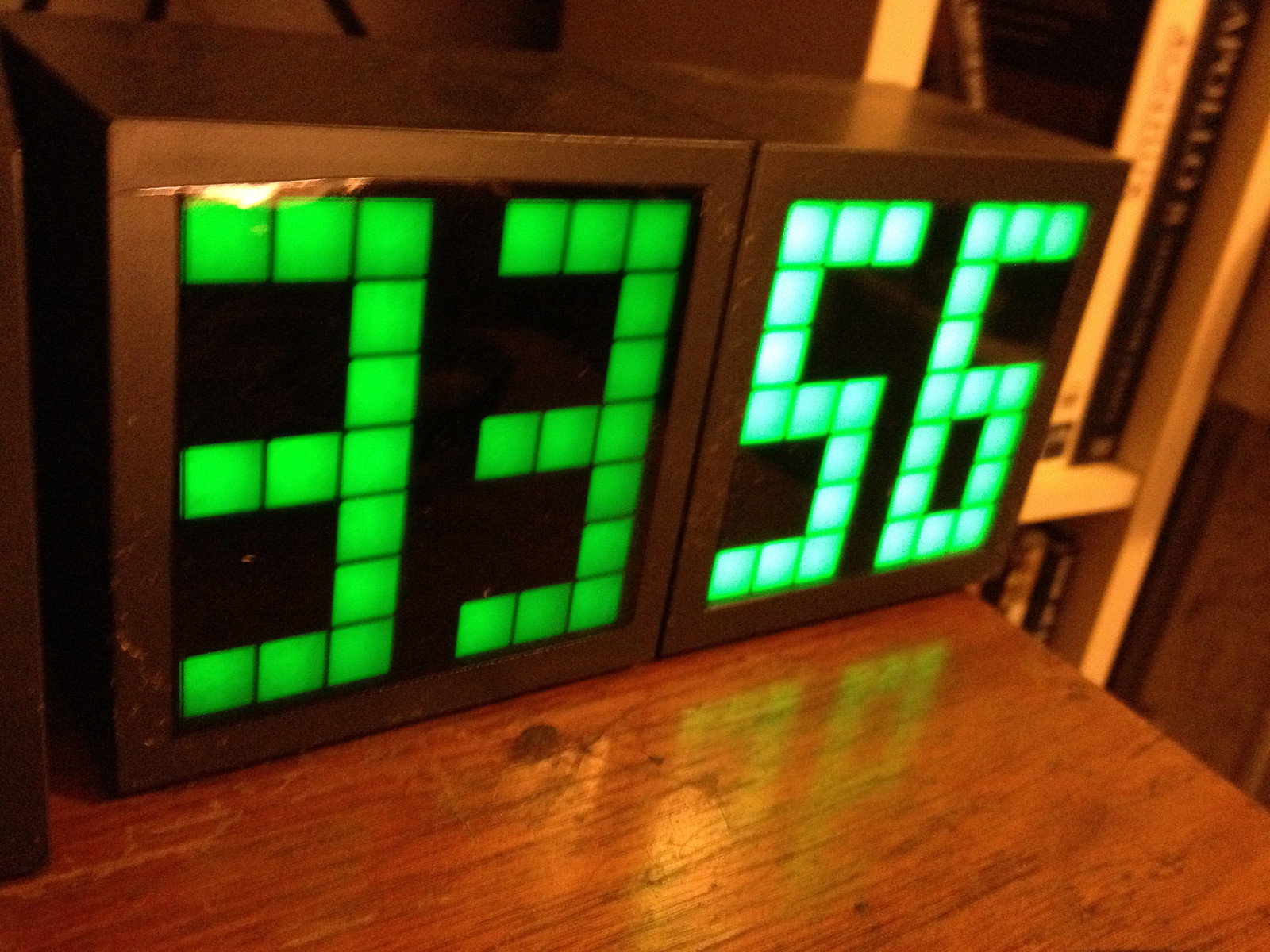In this detailed image, a dark brown weathered wood countertop or tabletop serves as the setting. On this surface rest two identical black, cube-shaped boxes with digital displays in their centers. The left box features a black square with a digital display that glows green, forming the numbers "33" from several small square-shaped tiles. Similarly, the right box also has a black background with a green digital display, here showing the numbers "56" with more illuminated tiles. The numbers appear in a block-like fashion reminiscent of Tetris pieces. To the right, in the background, a light wood or white bookcase is visible, adorned with a mix of books arranged both horizontally and vertically on its shelves.